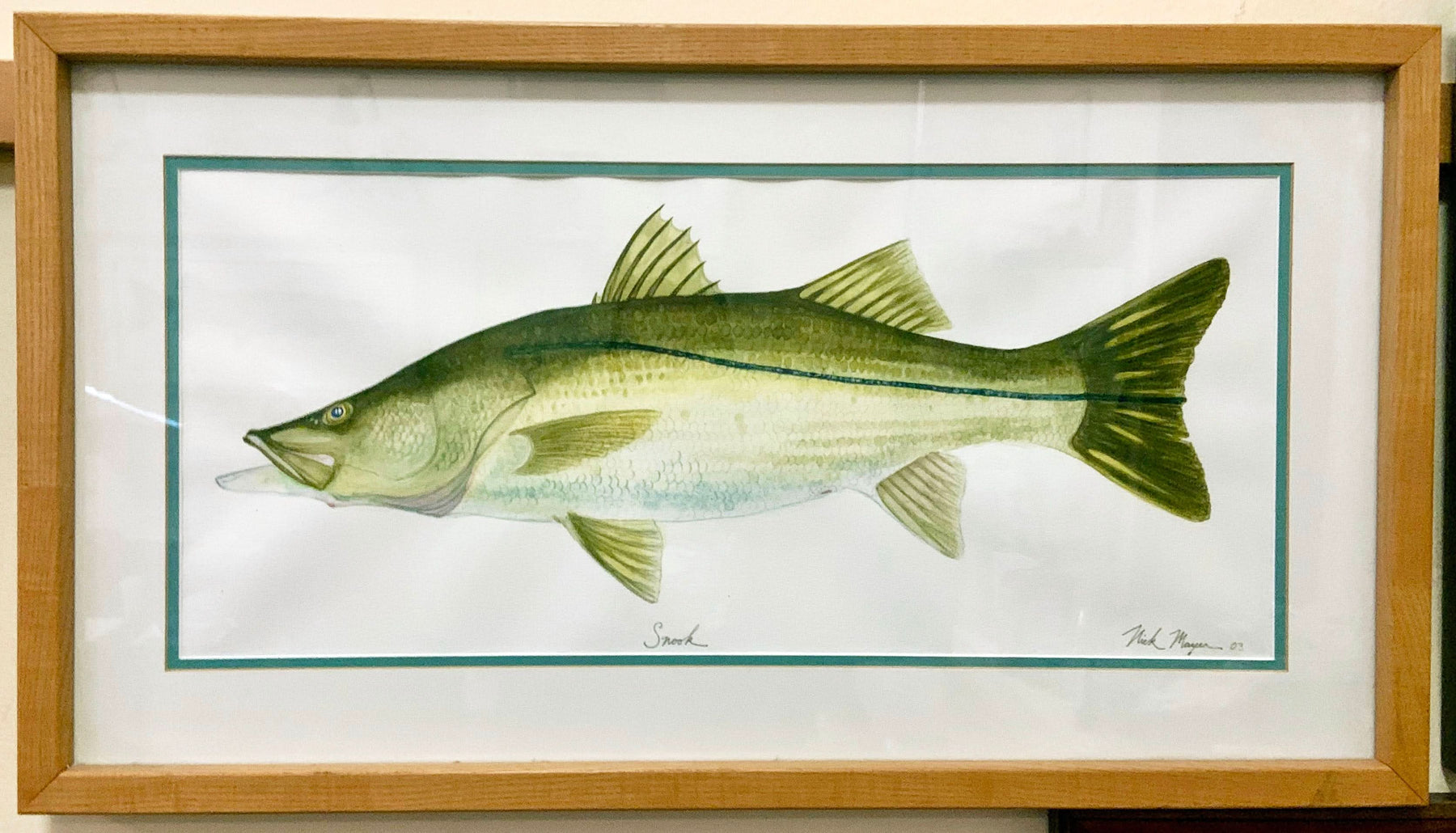This framed artwork showcases a hand-drawn image of a fish, specifically what appears to be a bass. The artwork is enclosed in a rectangular, light brown wooden frame that is oriented horizontally, with the top and bottom edges longer than the sides. Surrounding the image is a white mat adorned with a light green trim. 

The fish, viewed from the side, is predominantly green, featuring scales and fins with varying shades. The upper part of the fish is mostly dark green, fading into lighter green and white towards the belly. The fish's tail is positioned to the left, while the head, including a bluish eye, faces the right. The image highlights various fins: two on the top, two on the bottom, and one near the mouth. 

Below the fish, there appears to be a small, unreadable name, possibly identifying the fish as a snook, though the letters are too small to confirm. In the bottom right corner of the artwork, under the green outline, is an unreadable artist's signature. The piece is noted to have some mounting issues, with parts of the artwork bowing and appearing uneven within the mat.